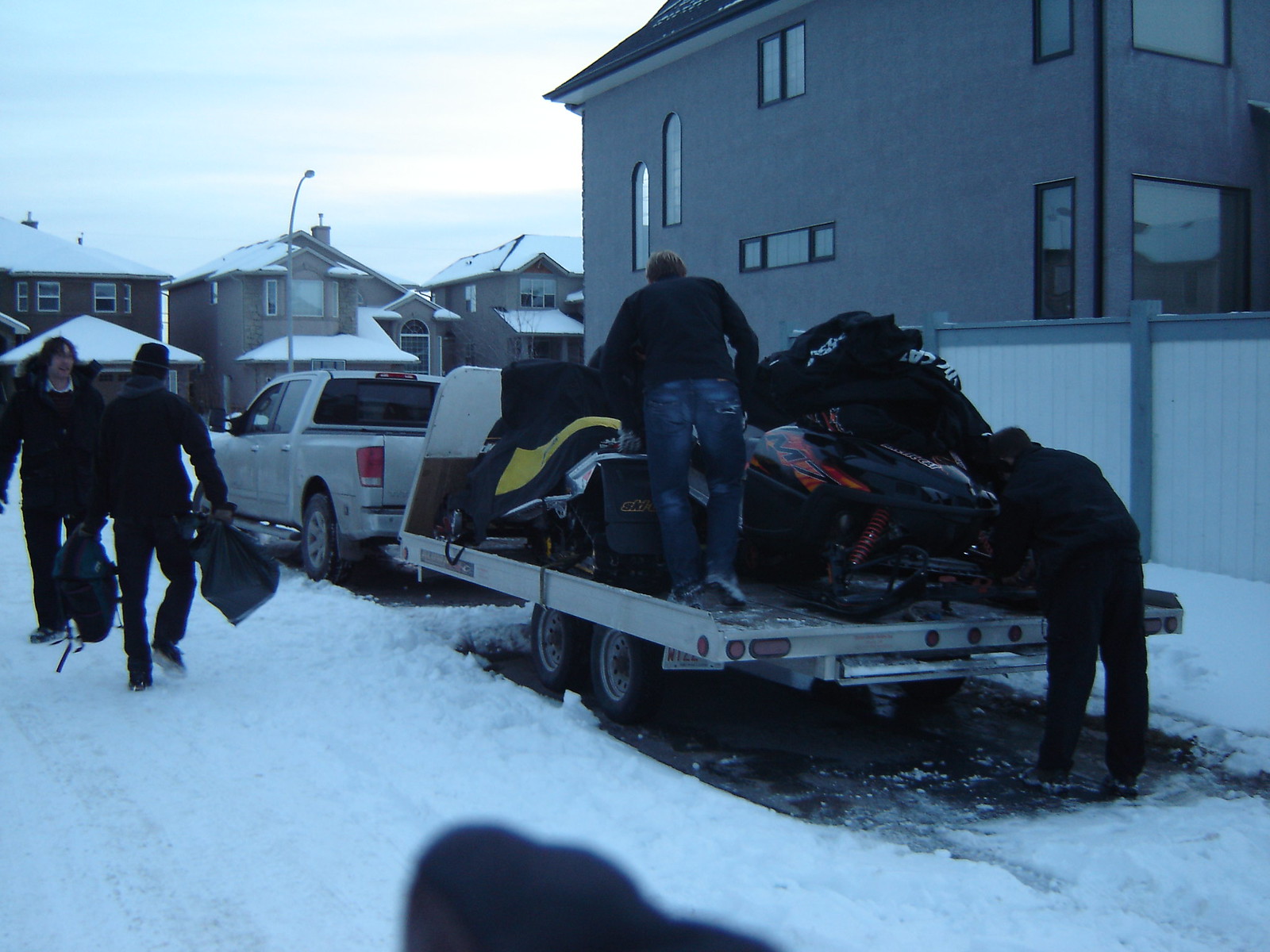In this detailed photograph, a scene unfolds in a snowy residential neighborhood where a group of men is preparing for a trip. The focal point is a Chevrolet pickup truck hitched to a flatbed trailer. The truck and trailer are parked on a driveway, with snow covering the ground around them, save for the areas immediately surrounding the vehicles, which have been shoveled clear. The trailer is densely packed with luggage, equipment, and possibly a snowmobile or two, secured under a tarp and some clothing.

Four men are actively engaged in the preparation: two are on the trailer, meticulously securing a snowmobile, while the other two men, clad in black thick winter coats, are on the left side of the scene. These two men are walking with backpacks and bags in hand, likely heading towards the truck to load more items. The early morning or overcast light gives a serene, almost cold ambiance to the photograph, contrasting with the energetic hustle of the men as they ready themselves for their journey against the picturesque backdrop of snow-covered houses.